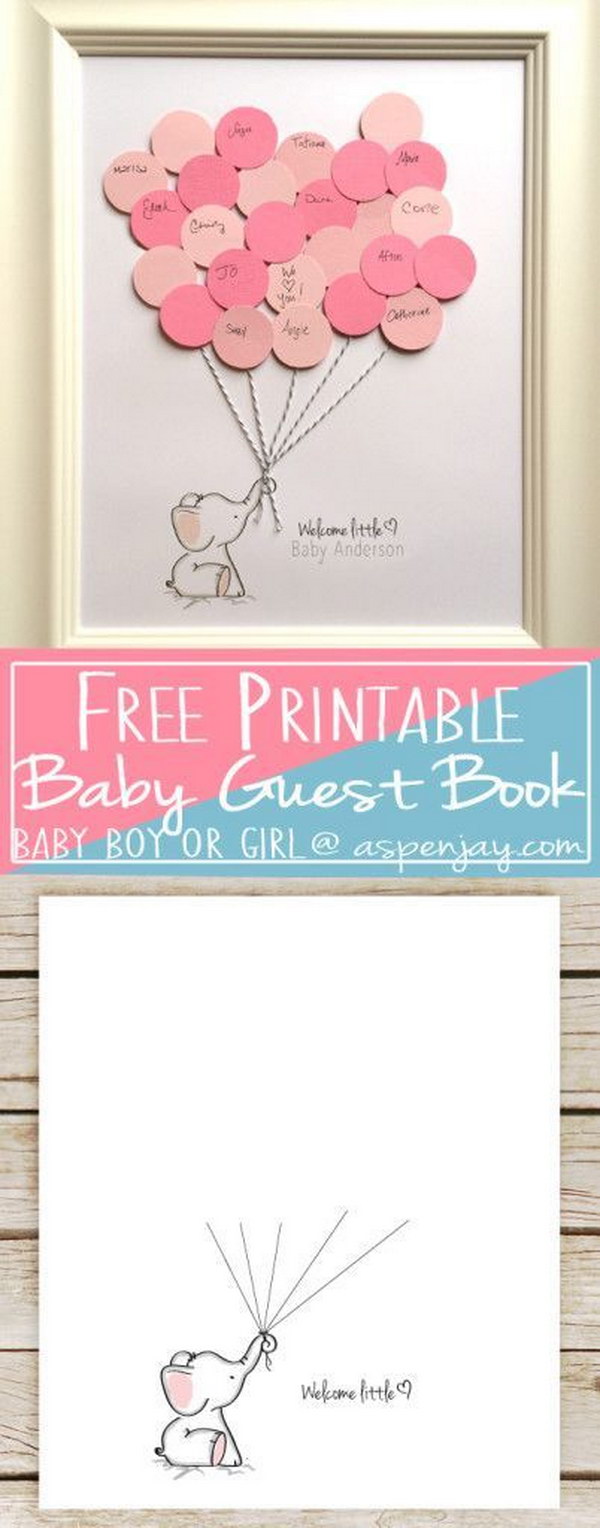This image is a detailed advertisement for a free printable baby guestbook available at AspenJay.com. It showcases a graphic design divided into three sections. The top section highlights the finished product, which features a shiny, cream-colored, beveled picture frame containing a charming illustration of a baby elephant. The elephant, painted with its trunk raised, holds five strings made of real string, each ending in a pink cardstock circle acting as balloons. These circles come in various shades of pink and some already have names written on them, while others are left blank for guests to fill in. The text "Welcome Little ♥ Baby Anderson" is handwritten to the right of the elephant.

The middle section of the image contains a promotional banner with a white inset border. It reads, "Free Printable Baby Guestbook for Baby Boy or Girl" with the website address AspenJay.com. The design features a pink hue on the top left blending into a blue hue on the bottom right, with white text overlaying the colorful background.

The bottom section displays the base artwork, showing the same baby elephant with its trunk raised and strings trailing upward but without any cardstock balloons attached. This illustrates how the design appears when first printed, ready for personalization by adding the paper balloons. A signature is visible to the right of the elephant in both the top and bottom framed pictures.